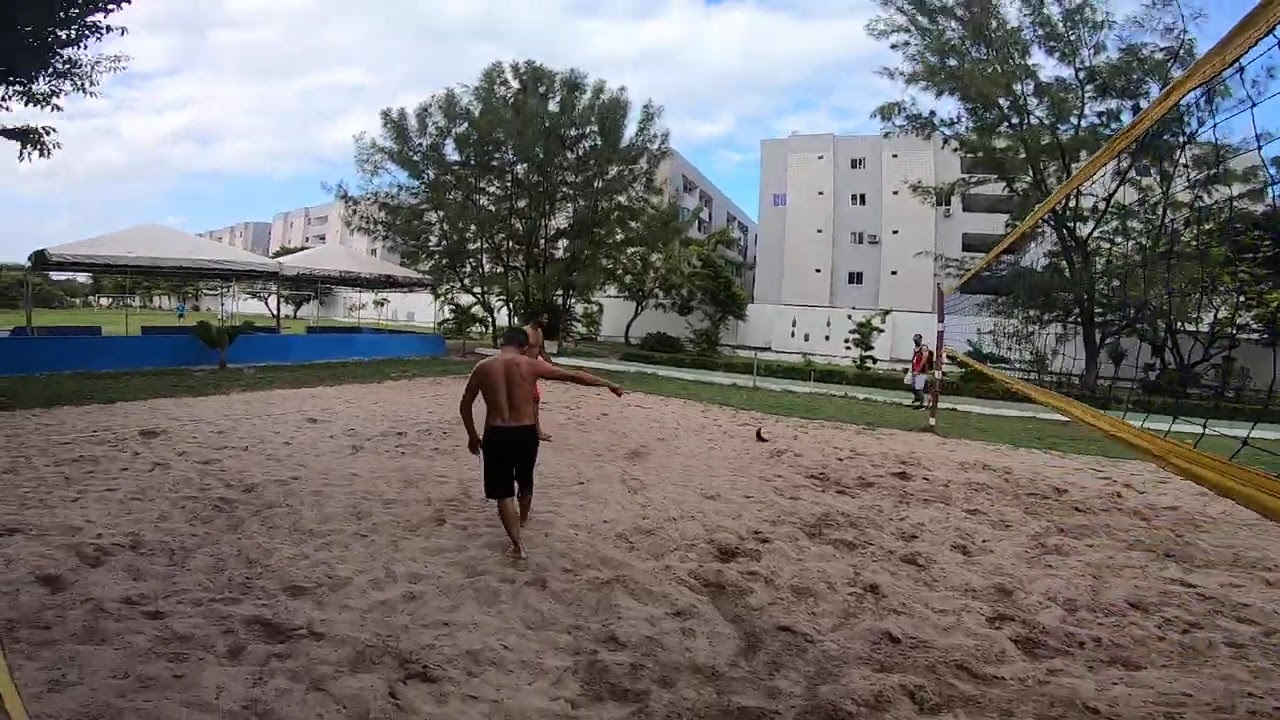In the image, there is an active beach volleyball game taking place in a sand court, distinguished by numerous footprints. The volleyball net, featuring yellow borders and black netting, divides the visible left half of the court, while the right half is obscured from view. Two young men, both shirtless and wearing black shorts, are visible on the court; one, positioned closer to the foreground, is facing away, pointing to the right with his right arm, while his left arm hangs by his side. The other player, partially obscured in the background, appears to be wearing red shorts. Sitting in the middle near the net, a third individual seems to serve as a casual referee. Surrounding the court, there's a grassy area with a couple of pavilions featuring white tops, and a blue fence partially enclosing the scene. The background includes several trees and a series of four- to five-story white buildings, possibly hotels or apartment complexes, characterized by small rectangular windows and potential steam vent openings. Further back, blue squared pyramid domes hint at a possible audience area. The sky above is overcast with numerous clouds, though it remains a bright day.